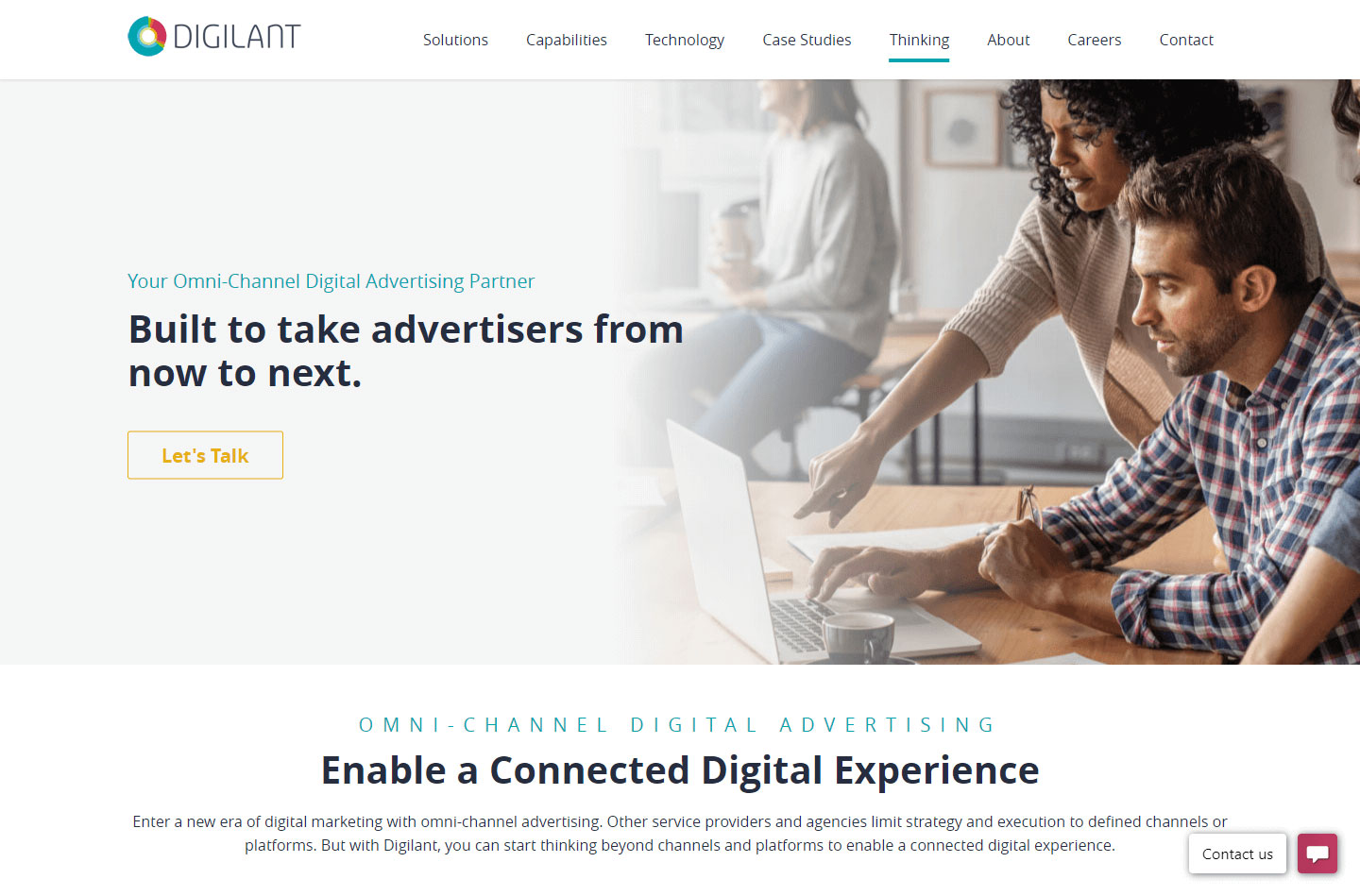In the upper left corner, the logo is displayed as a circle, composed of one-third red and two-thirds green. Adjacent to the logo, there are several navigation tabs labeled: Solutions, Capabilities, Technology, Case Studies, Thinking, Careers, and Contacts. Below these tabs, the main section features an image of a group in a modern office setting. A woman is prominently seen pointing at a laptop, while a man beside her writes down notes and clicks on the laptop.

To the left of the image, there is blue text reading "Your omni-channel digital advertising partner," followed by black text stating "Built to take advertisers from now to next." Beneath this text, a yellow button is prominently displayed with the call to action "Let's Talk."

Further down, additional text in a blue-green shade states "Omni-channel digital advertising," followed by black text that says "Enabled a connected digital experience." Below this description, more detailed information is presented: "Enter a new era of digital marketing with omni-channel advertising. Other service providers and agencies limit strategy and execution to defined channels or platforms. But with Digilent, you can start thinking beyond channels and platforms to enable a connected digital experience."

To the right of this text, there is a box labeled "Connect Us," and adjacent to it is a pink box featuring a white chat bubble.